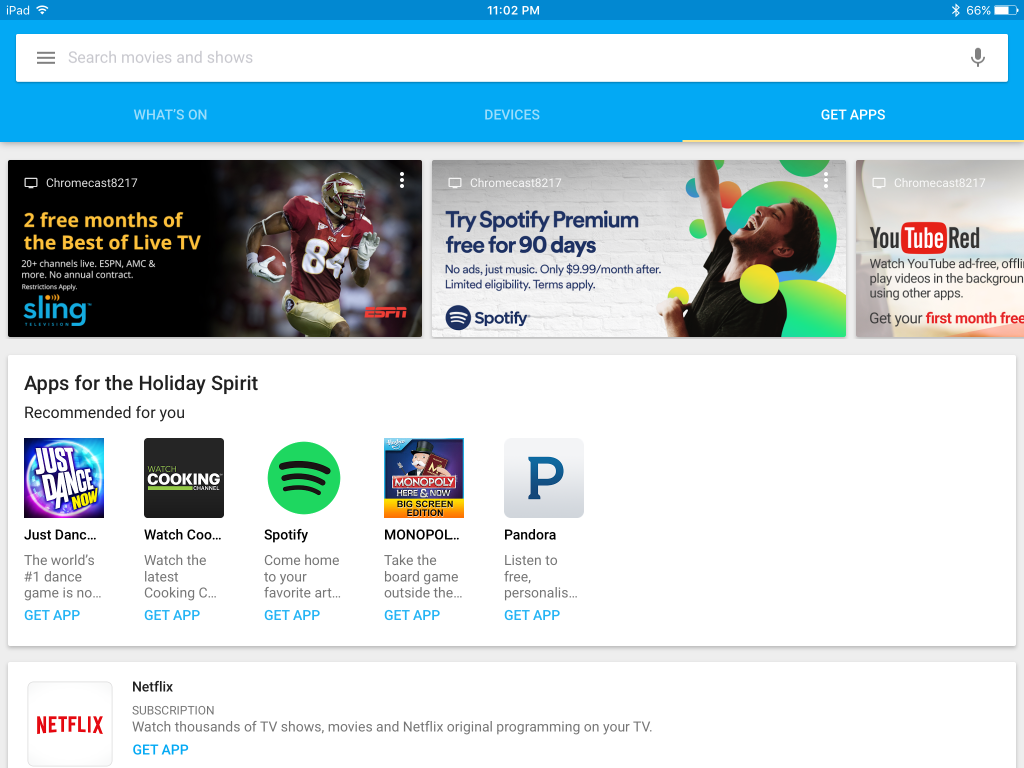A detailed close-up screenshot of a mobile device is displayed, primarily highlighting the device's app store interface. At the top of the screen, a bright blue header houses a white search bar. Above this bar, the time reads "11:02 PM." To the right of the search bar is the battery charge status, indicating a charge level of either 65% or 66%. On the top left side, there is a Wi-Fi icon and an unreadable word.

Below the search bar, three selectable options are visible: "What's New," "Top Devices," and "Get Apps." The screen then transitions into a section featuring sponsored advertisements. The first ad promotes Sling TV, offering "two free months of the best live TV" and highlighting ESPN with a football player image. The second ad offers a trial for Spotify Premium, free for 90 days, featuring a vibrant image of a person singing surrounded by colorful bubbles. The third ad advertises YouTube Red, offering the first month free.

Under the ads, a large white text box with bold lettering reads, "Apps for the Holiday Spirit Recommended for You," showcasing five applications: Just Dance, Cooking Channel, Spotify, Monopoly, and Pandora. Each app has a brief description:

- **Just Dance Now:** Touted as "The world's number one dance game."
- **Cooking Channel:** Encourages users to "Watch the latest cooking shows."
- **Spotify:** Suggests users "Come home to your favorite artist."
- **Monopoly:** (No visible description in the text)
- **Pandora:** (No visible description in the text)

Each app features a blue "GET APP" button in capital letters, inviting users to download.

A gray bar underneath separates this section from the next white text box dedicated to Netflix, which states, "Subscription: Watch thousands of TV shows." The invitation to "Get the Netflix app" is also present, but the content is cut off at this point.